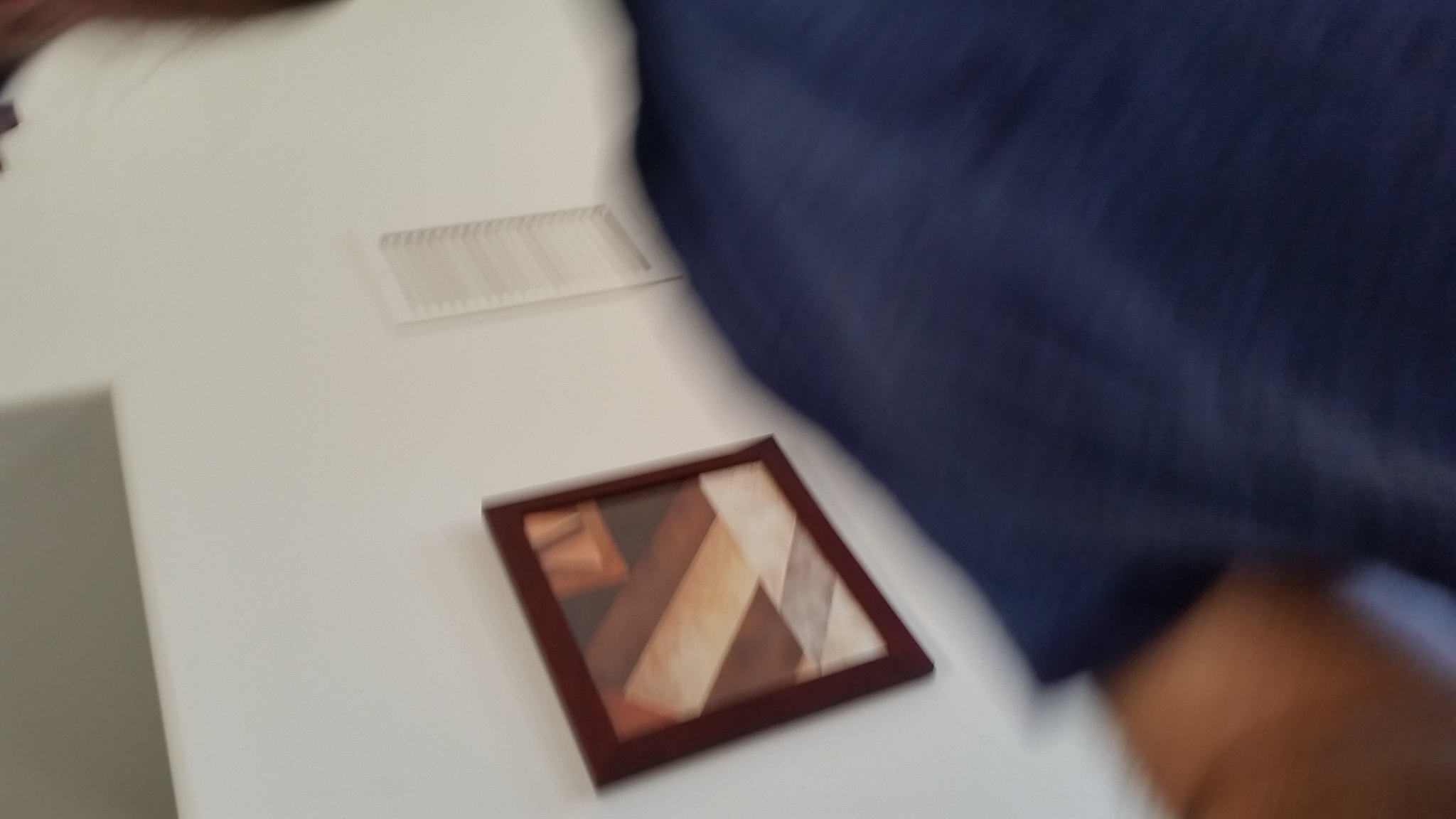The photograph appears to be an accidental upward-angle selfie of a person wearing a shiny blue, short-sleeved t-shirt. Their right arm is bent at the elbow and extends to the bottom right corner of the image, suggesting they are holding the camera in the palm of their hand. The person is almost horizontal in the frame, with some strands of their brown hair visible in the upper left corner. The background features a very bright white wall, with a heating and air conditioning vent near the top, almost at door height. To the left of the vent, there's a gray, darkened area resembling an open doorway or hallway. Centered on the wall is a square piece of art with a brown frame, which appears to be a print or painting. The artwork consists of geometrical shapes, with trapezoidal pieces in lighter gray, cream, brown, and beige, reminiscent of a tangram puzzle. The image captures a slightly distorted view of both the person and their surroundings, giving it a blurred, out-of-focus quality.